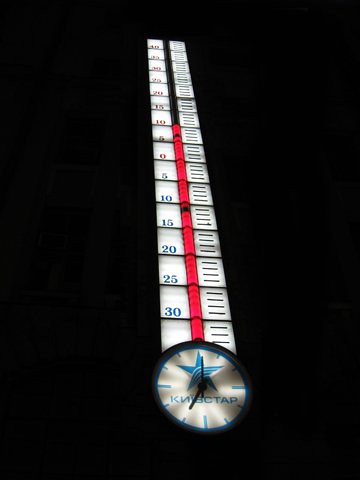This photograph captures an outdoor sign prominently displayed against a black background. The focal point of the image is a large, illuminated device that serves dual functions of displaying both the time and the temperature. 

At the base of the sign, a circular black disk houses a white clock face, indicating the time as approximately 11:35 PM. Above the clock face, a star can be seen inside the black circle, and a Russian word is inscribed beneath it.

Extending upwards from the clock, the sign features a vertical thermometer. This thermometer is uniquely detailed, with temperature markers ranging from -30 to +40 degrees Celsius. Each 5-degree increment is clearly marked by a rectangle, and more specific measurements are indicated with individual lines for each degree in-between, such as 31, 32, 33, and 34. The thermometer rises incrementally, with the rectangles continuing up the length of the sign to display the temperature clearly.

In the center of the thermometer, a red light indicator marks the current temperature. This well-lit, graphic display bears resemblance to the type of time and temperature signs often found outside banks in the United States but is notably more elaborate in its presentation and scale.